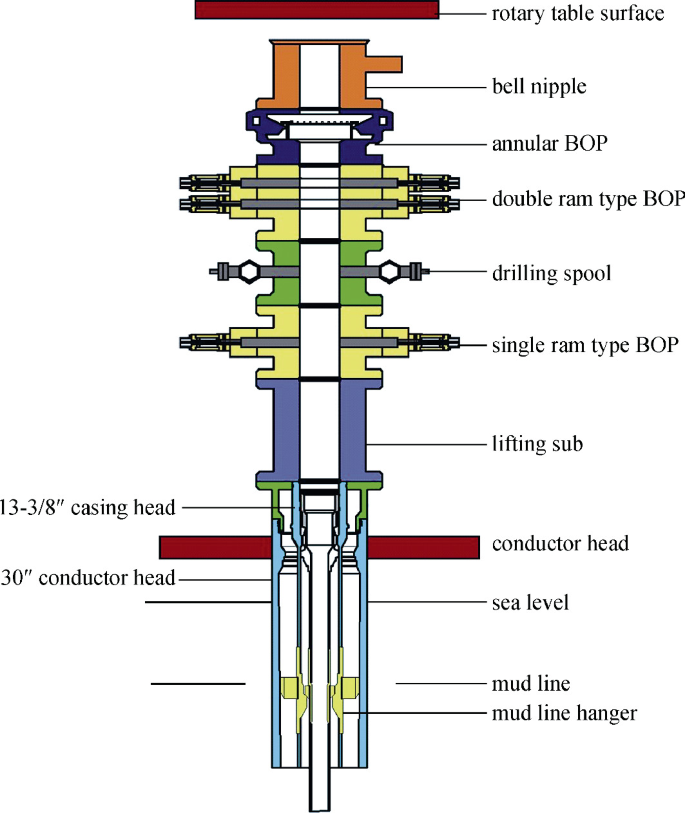This is a detailed, vertical rectangular schematic illustration of an underwater drilling rig. The color-coded diagram meticulously labels each component with lines connecting to their respective labels. At the top, a small red rectangle labeled "rotary table surface" marks the beginning of the structure. Below it, successive components include the "bell nipple," "annular BOP," "double ram type BOP," "drilling spool," "single ram type BOP," and "lifting sub," which is colored purple. Moving further down, the diagram identifies the "13 3/8 casing head" on the left and the "conductor head" alongside the "30 inch conductor head." Critical reference points such as "sea level" and "mud line" are clearly indicated, with multiple instances of "mud line hanger" labeled for emphasis. This comprehensive color illustration serves as a detailed reference guide to the intricate parts and structure of a deep-water drilling system.